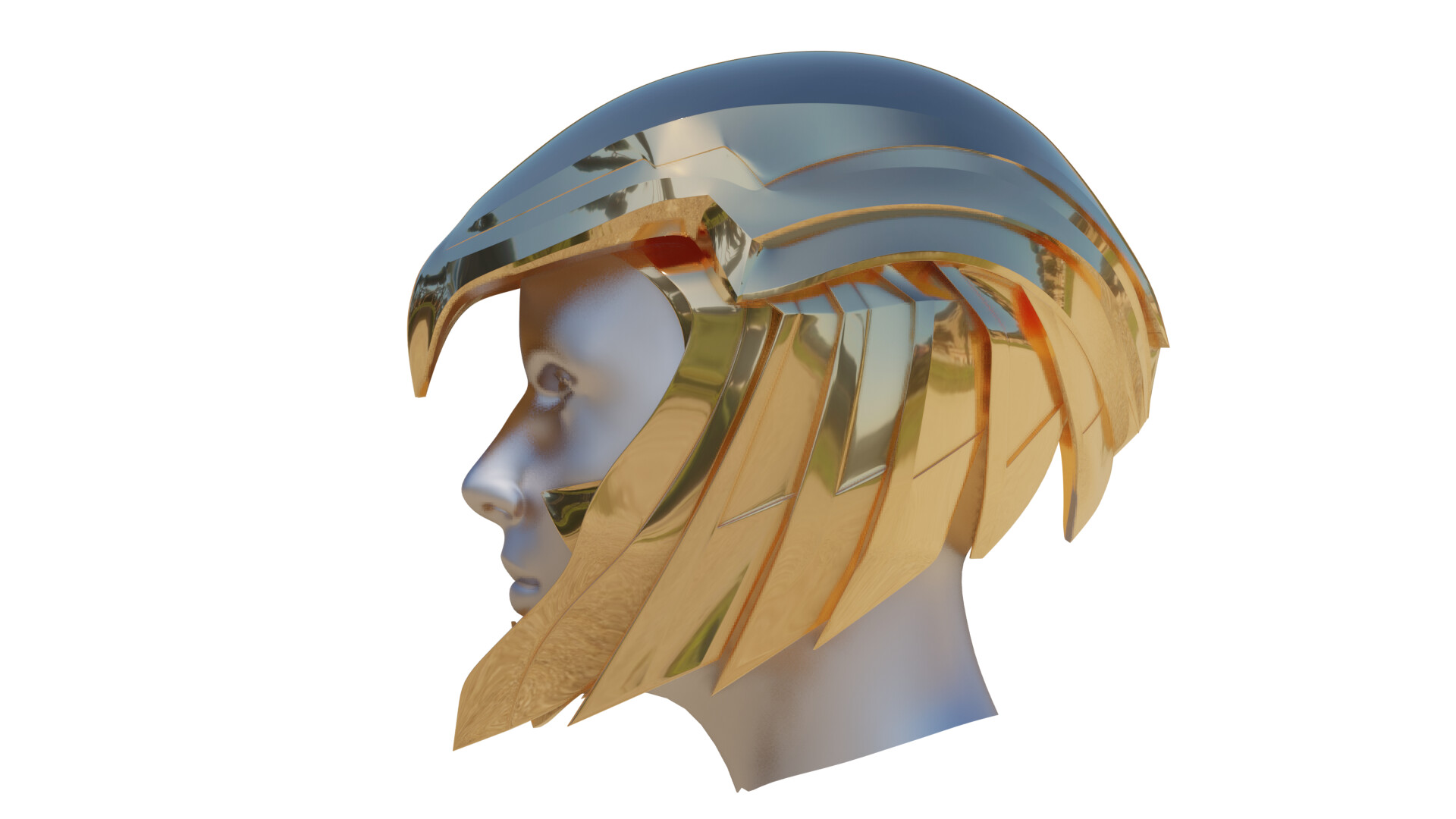The image is a digital screenshot of a 3D render featuring a plaster-like mannequin head adorned with a uniquely shaped blue helmet designed to resemble an eagle's head. The beak of the helmet is positioned directly in front of the eyes, while the sides of the helmet are embellished with shiny, gold-colored feathers that evoke an eagle's wings. The head is turned to the left, revealing the intricate details of the helmet's design against a white background. The scene prominently displays shades of blue, gold, silver, and additional hues like orange, white, gray, and green, creating a striking and detailed visual.